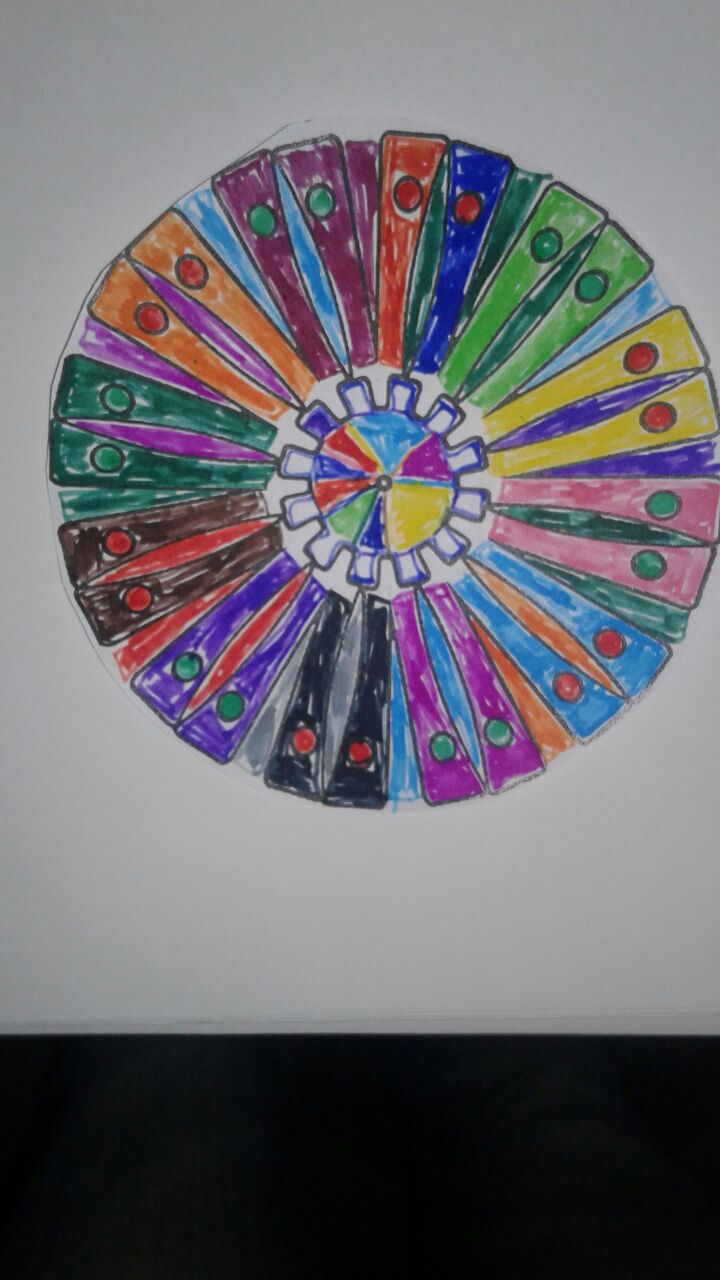This detailed drawing, set on a piece of white paper in a rectangular portrait orientation, features a striking arrangement of piano keys creatively reimagined in a circular formation. Vibrantly colored keys—ranging from shades of burgundy, green, orange, red, blue, yellow, purple, and pink—encircle the composition. Each set of keys, grouped in pairs, is distinctively colored both in the key and the circular design at its center, creating a kaleidoscopic visual effect. A solid black bar at the bottom of this image anchors the dynamic hues of the circular piano keys above, adding a stark contrast that enhances the overall aesthetic appeal.